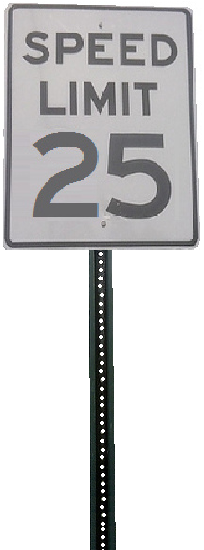The image depicts a speed limit sign mounted on a dark-colored metal pole. The overall style of the photograph appears somewhat blocky and partially rendered, giving it an unfinished look. The metal pole features small circular indentations running vertically along its length. The speed limit sign itself has an off-white background with a gray border. The text on the sign is in uppercase letters, stating "SPEED LIMIT" above the number "25" in gray. Both the top and bottom of the image show circular brackets where the sign is attached to the pole. The image exhibits a degree of sloppiness, with visible blurring effects in certain areas, contributing to its overall blocky appearance.